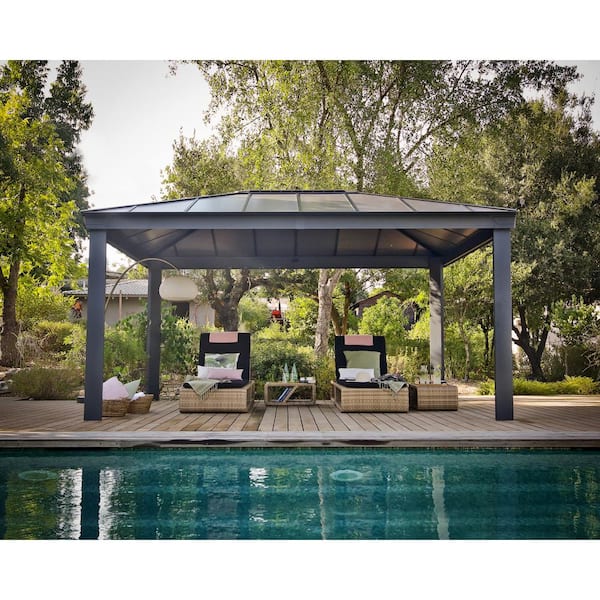This image captures an idyllic outdoor pool lounge area on a pleasant summer day. In the forefront, the serene turquoise water of the swimming pool reflects the tranquil atmosphere. Adjacent to the pool lies a wooden deck made of pale, teak-like planks. Atop the deck sits a shaded pergola with metal posts and a brown-topped canopy providing shade to two wicker lounge chairs. These tan wicker chairs, equipped for ultimate relaxation, feature plush black cushions, adorned with light pink towels draped over their backs and various pillows, including beige ones behind smaller white pillows. Between the lounge chairs is a matching wicker side table, hosting a couple of bottles, likely containing refreshing drinks. Another small wicker table is positioned beside one of the loungers. The background reveals a lush scene of trees and bushes, enhancing the serene ambiance, with a glimpse of a low, flat house partially hidden behind the greenery. The sky is gray, and the overall setting reflects a perfectly manicured and inviting summer retreat.